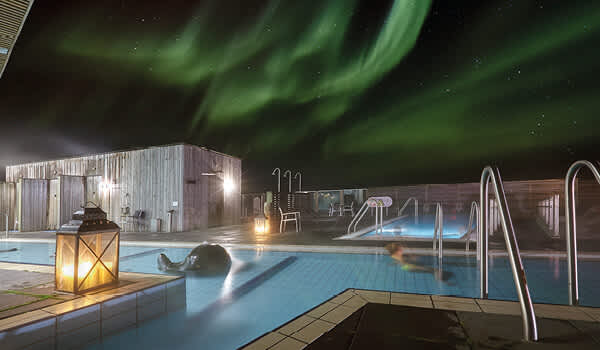The image depicts a nighttime scene with a breathtaking display of the northern lights illuminating the sky in green wisps, interspersed with visible stars. The perspective is horizontal, showing a rooftop setting that includes a serene swimming pool filled with transparent water. The pool is T-shaped, with the base starting at the lower left corner and extending diagonally to the right before forming the top of the T. To the left of the pool, a wooden building with two open doors is visible, and a lantern is positioned on the deck near the corner of the pool. In the shallow end of the pool, there is a black fountain feature. Adjacent to the main pool is a smaller rectangular pool, possibly a hot tub. A single, blurry figure, likely a woman, is in the main pool near a ladder on the right side. The overall ambiance is serene and somewhat mysterious, highlighted by the interplay of natural and artificial lighting.